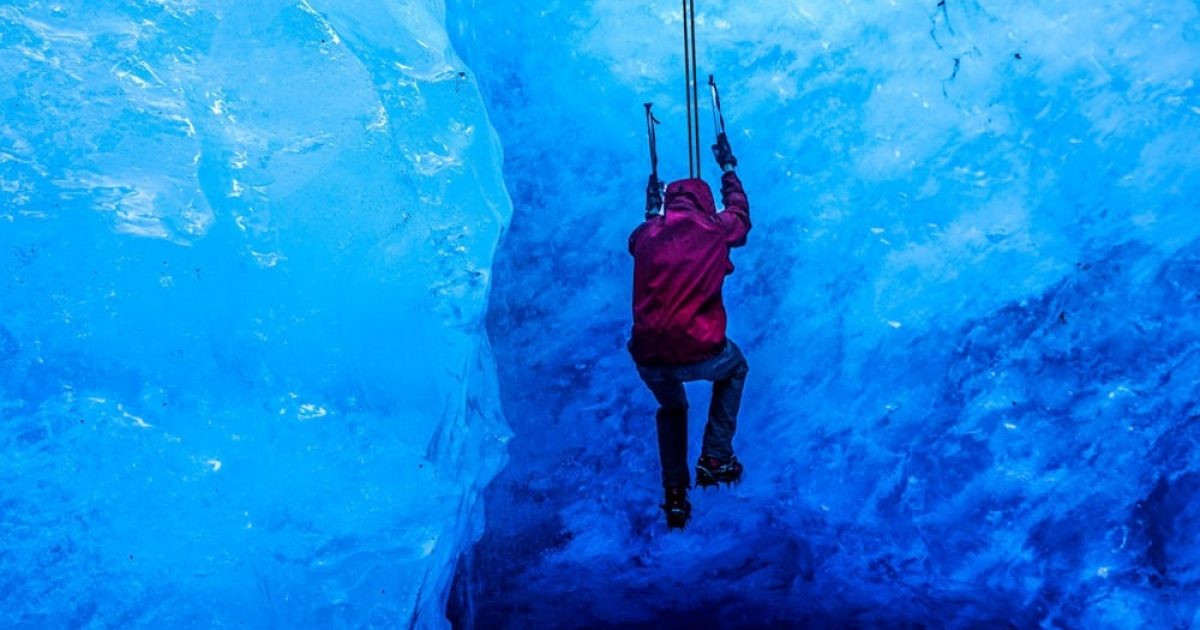In this captivating photograph, a man clad in a striking red jacket and blue pants is seen ice climbing against a stunningly textured icy blue surface, possibly a glacier. The climber, whose face is hidden beneath the hood of his jacket, is equipped with specialized gear, including spiked shoes for traction and black gloves gripping two ice picks embedded in the ice above his head. He is securely fastened with a safety line and cables, suggesting the formidable and treacherous nature of his ascent or descent. Surrounding him is a mesmerizing landscape of varying shades of blue and white ice, adding to the eerie yet awe-inspiring atmosphere of the scene. The vivid contrast between the climber's attire and the glacial background adds a dramatic element, capturing the essence of the chilly, adventurous endeavor.